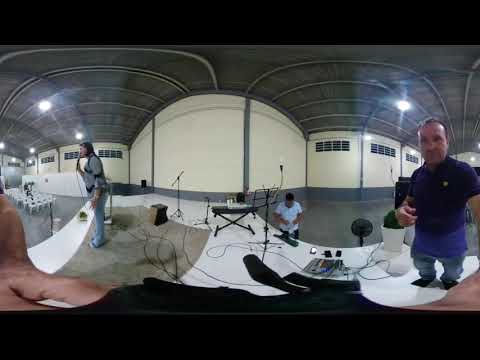This image depicts the scene inside a large indoor space, potentially a warehouse or hangar, characterized by its rounded white walls and dark gray, arched ceiling with double rainbow-like lines. At the top and bottom of the image, a solid black border frames the view. The setting includes concrete flooring and several pieces of musical equipment, suggesting a setup for a sound test or musical performance.

In the center of the image, the musical instruments are prominently positioned. A keyboard is visible, accompanied by a music stand and several microphones. There are also numerous pieces of electrical equipment and wires scattered around, enhancing the impression of a preparation for an event.

Three individuals are present in the picture. On the right side, a man stands close to the camera, facing directly towards it. He is balding and wears a dark blue polo shirt paired with blue pants. His right arm appears to be holding something, possibly related to the equipment around him. To the left, another person stands holding a microphone, wearing a gray shirt and light blue pants, and facing left. Near the lower center of the image is a third man, dressed in a white T-shirt and dark-colored pants, looking downward.

The backdrop includes gray ceiling lines and black windows at the top of the walls, adding to the industrial feel of the location. No text is visible in the image, and the color palette features black, white, gray, tan, green, and purple tones. The overall atmosphere suggests a moment of preparation in a spacious, indoor venue.